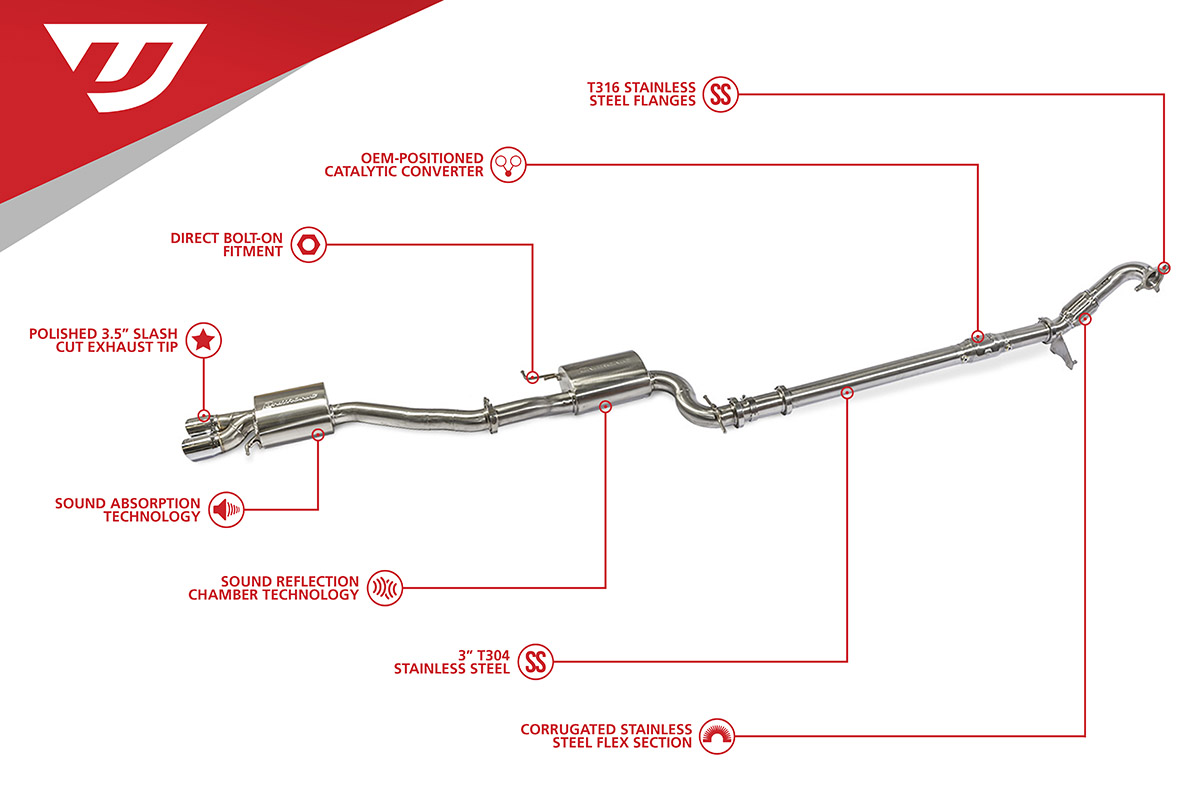The image features a detailed diagram of an exhaust system, showcasing a polished 3.5-inch slash cut exhaust tip. The diagram is set against a white background and includes a variety of components such as a muffler and a catalytic converter, which extends across the entire system from the engine attachment to the exhaust tip. The exhaust system is highlighted with several red lines pointing to labeled sections like the T316 stainless steel flanges, OEM-positioned catalytic converter, direct bolt-on fitment, sound absorption technology, sound reflection chamber technology, and corrugated stainless steel flex section. The diagram is visually marked at the top with a red triangle containing a white badge with a "U" on it, giving it a distinctive emblem. The red lines are accompanied by small icons depicting the function of each call-out, making it a comprehensive and visually descriptive overview of the exhaust system.